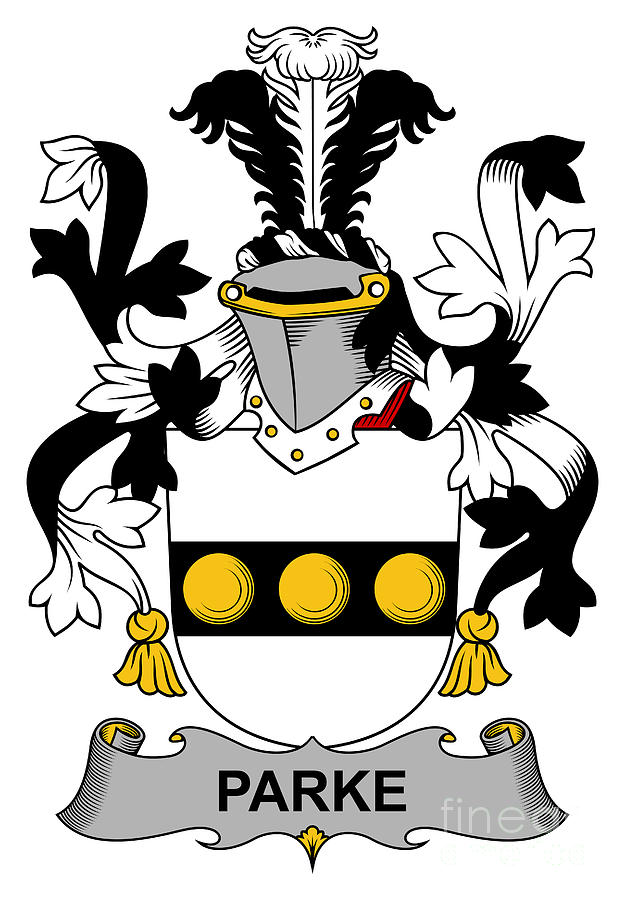This intricate black-and-white illustration features a detailed family crest on a white background with gold and gray highlights. Central to the crest is a shield marked by a horizontal black band embedded with three gold buttons. Above the shield perches a knight’s helmet with the visor down, accented by a small red detail at the base and golden embellishments. Emanating from the helmet are feathery extensions featuring a large central white feather flanked by black feathers. Black and white fleur-de-lis designs arch gracefully to the sides of the shield and helmet, adorned with dangling gold tassels. The name 'Parke,' highlighted in a sophisticated gray banner, anchors the bottom of the crest, adding an elegant touch to this meticulously crafted emblem.